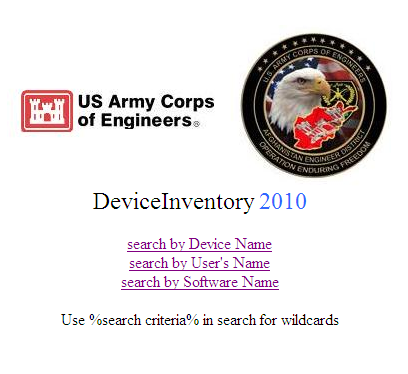The image is a screenshot of a web page with a predominantly white background that seamlessly blends into the rest of the screen. At the upper left corner is a small red square logo containing a white castle, representing the U.S. Army Corps of Engineers. To the right, in bold black text, it says "U.S. Army Corps of Engineers." In the upper right corner, there's a large circular emblem. This black circle features the text "U.S. Army Corps of Engineers" at the top and "Afghanistan Engineer District" at the bottom, with stars adorning the upper rim and "Operation Enduring Freedom" inscribed at the lower rim. Inside, it showcases a bald eagle in front of an American flag, further overlaid by the red outline of Afghanistan. Centered in the midline of the page is the header "Device Inventory 2010" in black and blue text. Below are three underlined links in a reddish-purple color, stating "Search by Device Name," "Search by User's Name," and "Search by Software Name." At the bottom, in black text, it reads "Use Search Criteria" and "Search for Wildcards." The colors used in the image are primarily black, white, red, tan, yellow, and dark blue.